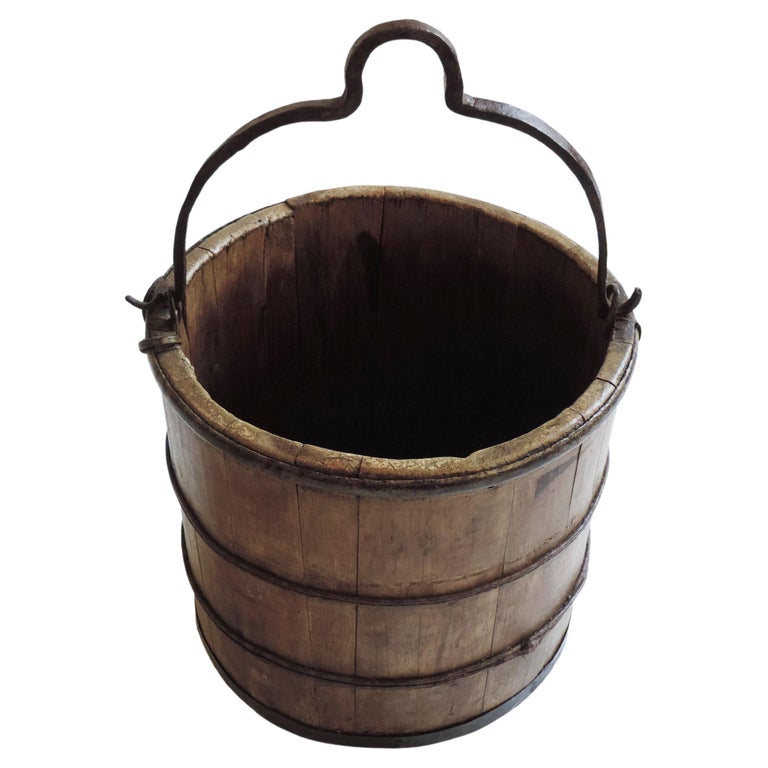The image depicts a reproduction of an antiquated wooden bucket against a solid white background, likely a product image. The bucket exhibits a hand-crafted, pioneer-era design, showcasing a basin formed from dark brown wooden slats held together by four metal rings—one at the top, two in the middle, and one at the bottom. Its structure bears a strong resemblance to a barrel, with a metal ring accentuating the bottom. The bucket has a deep interior, shrouded in shadow from the current lighting, ensuring the bottom remains unseen. At the top, a curved wrought iron handle is prominently featured. The overall composition emphasizes the bucket’s rustic and functional aesthetic, suitable for purchase, potentially sourced from a blacksmith shop.